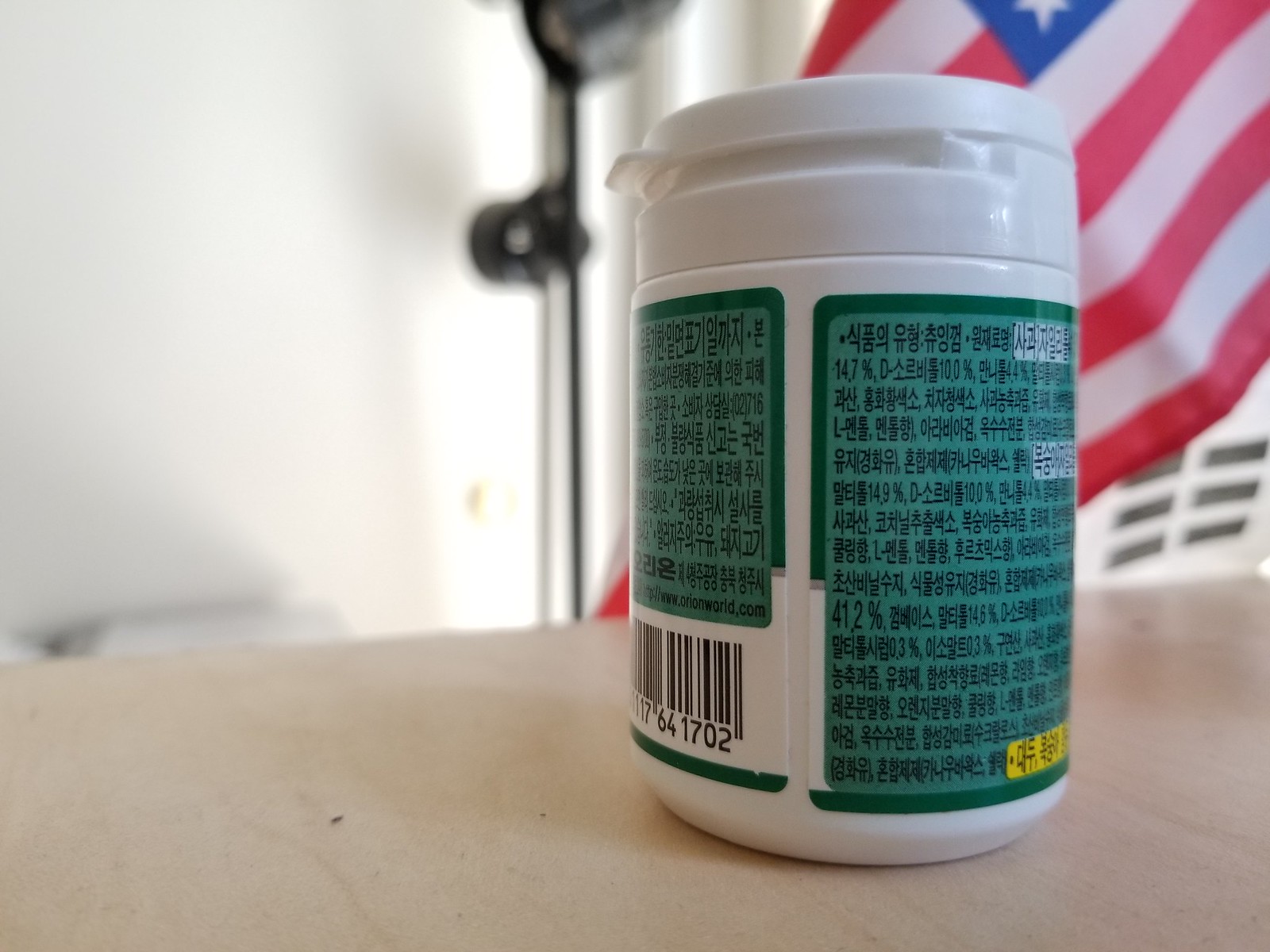This image is a horizontally oriented, up-close photograph of a small white plastic bottle with a flip-top lid, sitting on a light beige or cream-colored table. The bottle features green labels that are crowded with Chinese and Japanese writing, although the only discernible detail amidst the text is "41.2%." On the bottom left of the bottle is a white barcode with black lines. The background includes the red and white stripes and part of the blue section of an American flag, along with a black pole, possibly holding a fan, positioned just left of center. The upper left side of the photograph is white, indicating a wall or brightly lit area.